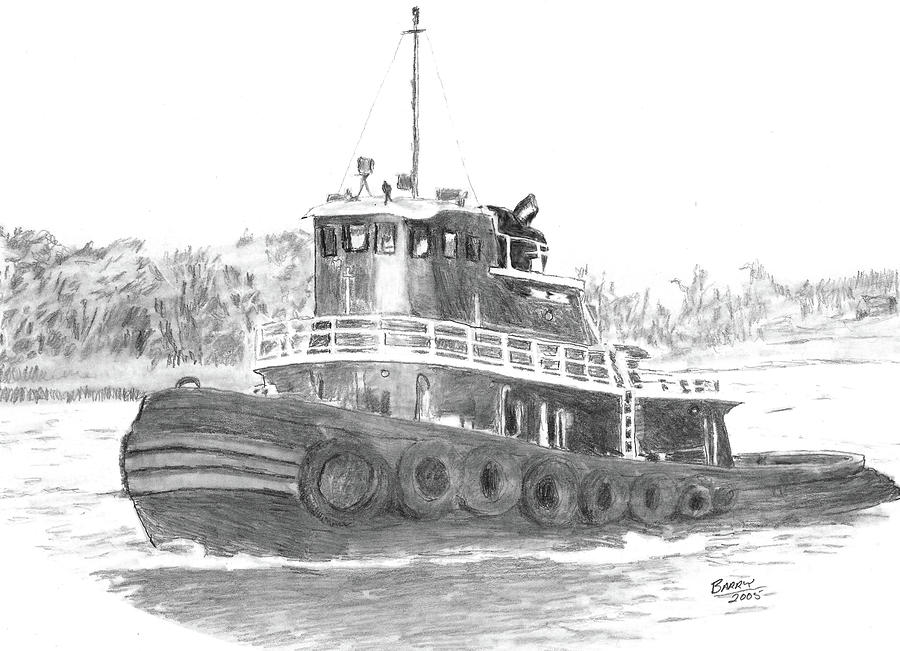The image is a black and white pencil drawing of a steamboat or tugboat on a river, signed Barry, 2005, in the bottom right corner. The boat, which spans approximately 50% of the drawing and is centered, is depicted in motion. It features a bowl-like shape, starting flatter at the back and curving upwards at the front. Along the right side of the boat are numerous tire-like flotation devices of varying sizes. The boat includes three tiers: the first tier supports many pillars, the mid-tier has a white railing, windows, and potentially the captain's quarters, and the top tier has radar, a mast with possible antennas and spotlights, and a large dark object shaped like an apple. 

In the background, the illustration shows sketchy trees lining the river and some etched plants along the river edge. The sky is left white, contrasting with the dark tone of the boat and the shaded water. Some additional details include a series of portholes, ladders, railings, and cables running across the boat. The person on the top level, though not detailed, implies human activity. The overall composition emphasizes the boat against the serene, natural backdrop of trees and river.